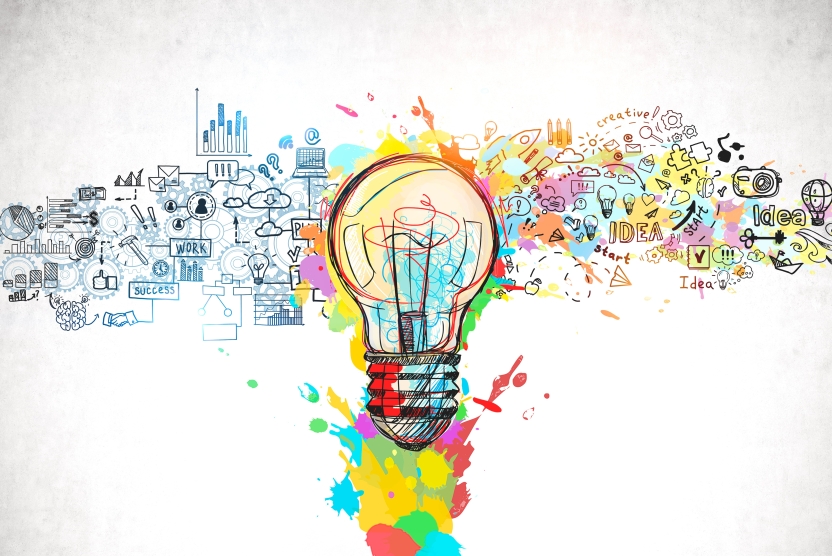The artwork poster is set against a stark white background. At the center lies an old-fashioned light bulb, its interior metal filaments visible and intricately detailed. This central light bulb symbolizes the birth of ideas, as if igniting a multitude of thoughts. Surrounding the base of the bulb are vibrant splashes of color—gold, aqua, green, and pink—spreading outwards.

On either side, the poster showcases numerous hand-drawn illustrations and objects, blending historical and contemporary ideas. To the left, features are predominantly in hues of blue and black, incorporating images like gears, charts, and a computer. On the right, the drawings burst with colors and depict items like hot air balloons, a radio, hands shaking, a music note, and puzzle pieces. Edward's idea, as well as words like "idea," "work," and "success," are interspersed throughout. The filament inside the bulb itself is a swirl of multiple colors—blues, reds—symbolizing creative spark. The colorful splashes and eclectic mix of images and words unify to create an intricate, vibrant depiction of collective human innovation and brainstorming, making the poster a rich tapestry of ideas and creativity.